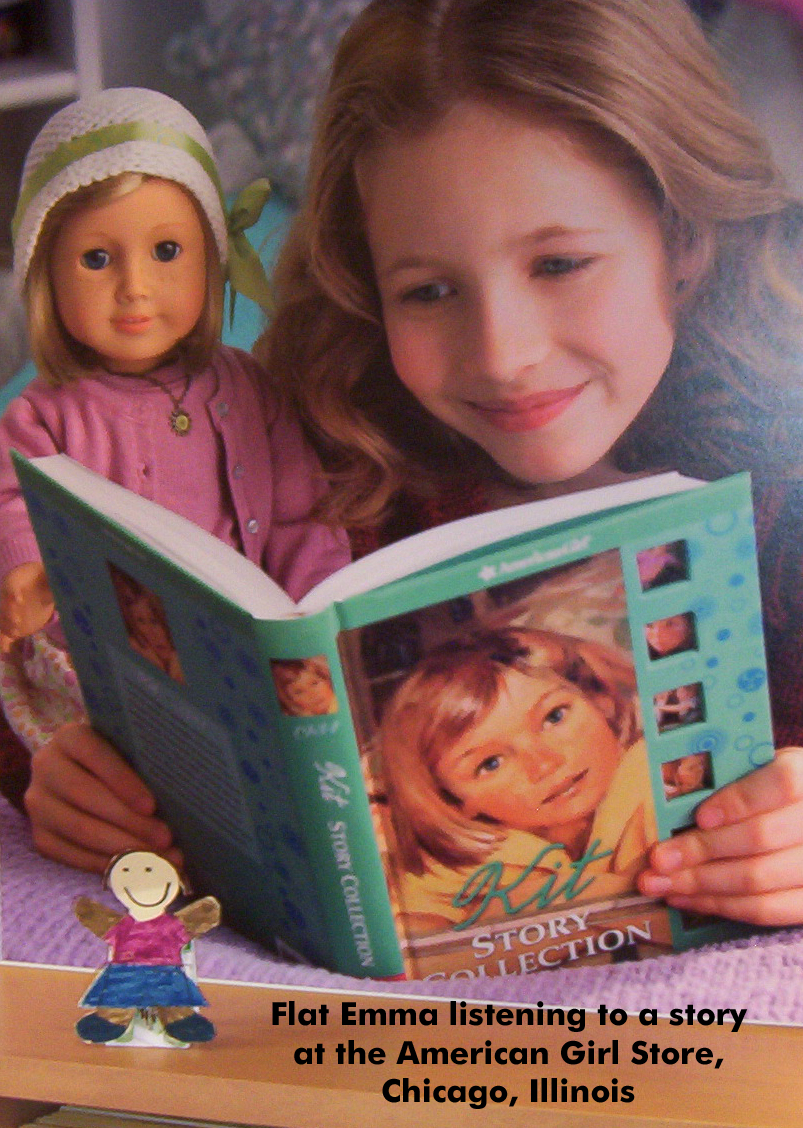The image is an advertisement from the 1990s, evidenced by the style elements such as the girl's wavy brown hair and the color palette. It depicts a young, light-brown-haired girl, likely a teenager, lying belly-first on a bed with a light purple mattress or cushion. The right side of the image shows a bit of glare, indicating it was a picture of a photo taken under natural lighting or room light. The room's background is blurred, revealing faint glimpses of walls or cabinets.

The central focus is on the girl, who is smiling while reading a hardcover book titled "Kit Story Collection." The book's teal cover features a picture of a young girl, and the title is printed vertically on the spine. The girl is holding the book with both hands, and sitting next to her right shoulder is a doll dressed in a pink cardigan and a white knitted hat with a green ribbon. The bed's wooden border, visible in the image, holds a cut-out of a child's drawing of a girl in a pink T-shirt and blue skirt, with black hands and a brown round head sporting a smiley face. Accompanying this illustration is a caption that reads "Flat Emma listening to a story at the American Girl Store, Chicago, Illinois."